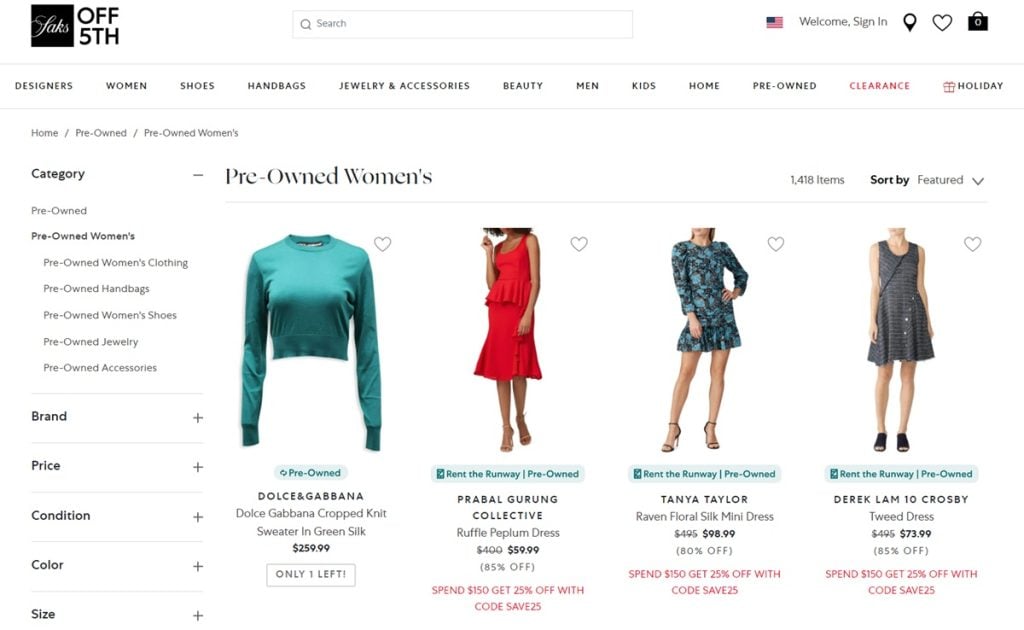This image captures a screenshot of the Saks Fifth Avenue website, showcasing its streamlined design and navigational elements. The background is predominantly white, which lends a clean, minimalistic feel to the interface. In the upper left-hand corner, the Saks logo is prominently displayed. Adjacent to the logo, in bold black capital letters, is the text "OFF 5TH."

Towards the center-right, a gray search bar is positioned for easy access. Further to the right, there's an American flag icon indicating the region, followed by a welcoming message in gray that reads "Welcome, sign in." Flanking this text are three icons: a shopping bag, a heart, and a map-like icon, presumably for cart, wishlist, and store locator functions, respectively.

Immediately below this header is the main menu bar, rendered in black text for high visibility. The menu categories include Designers, Women, Shoes, Handbags, Jewelry & Accessories, Beauty, Men, Kids, Home, Pre-Owned, and Clearance—rendered in red for emphasis. Nearby is the Holiday section, accompanied by a red gift icon for easy identification.

On the left side of the screen, a navigational breadcrumb trail in gray reads "Home / Pre-Owned / Pre-Owned Women's." Approximately two lines below, a vertical sidebar menu lists categories, starting with "Pre-Owned" and "Pre-Owned Women's," and extending to subcategories like Pre-Owned Clothing, Handbags, Shoes, and more. These subcategories can be expanded using gray plus signs to explore further by Brand, Price, Condition, Color, and Size.

At the top, to the right of the sidebar, the text "Pre-Owned Women's" is bold and underlined with a light gray line spanning the width of the screen. On the main portion of the screen, there are pictures of four clothing items displayed in a grid. The items include a green top, a red dress, a blue and black dress, and a gray dress. Each dress is detailed with its name and price directly beneath its image.